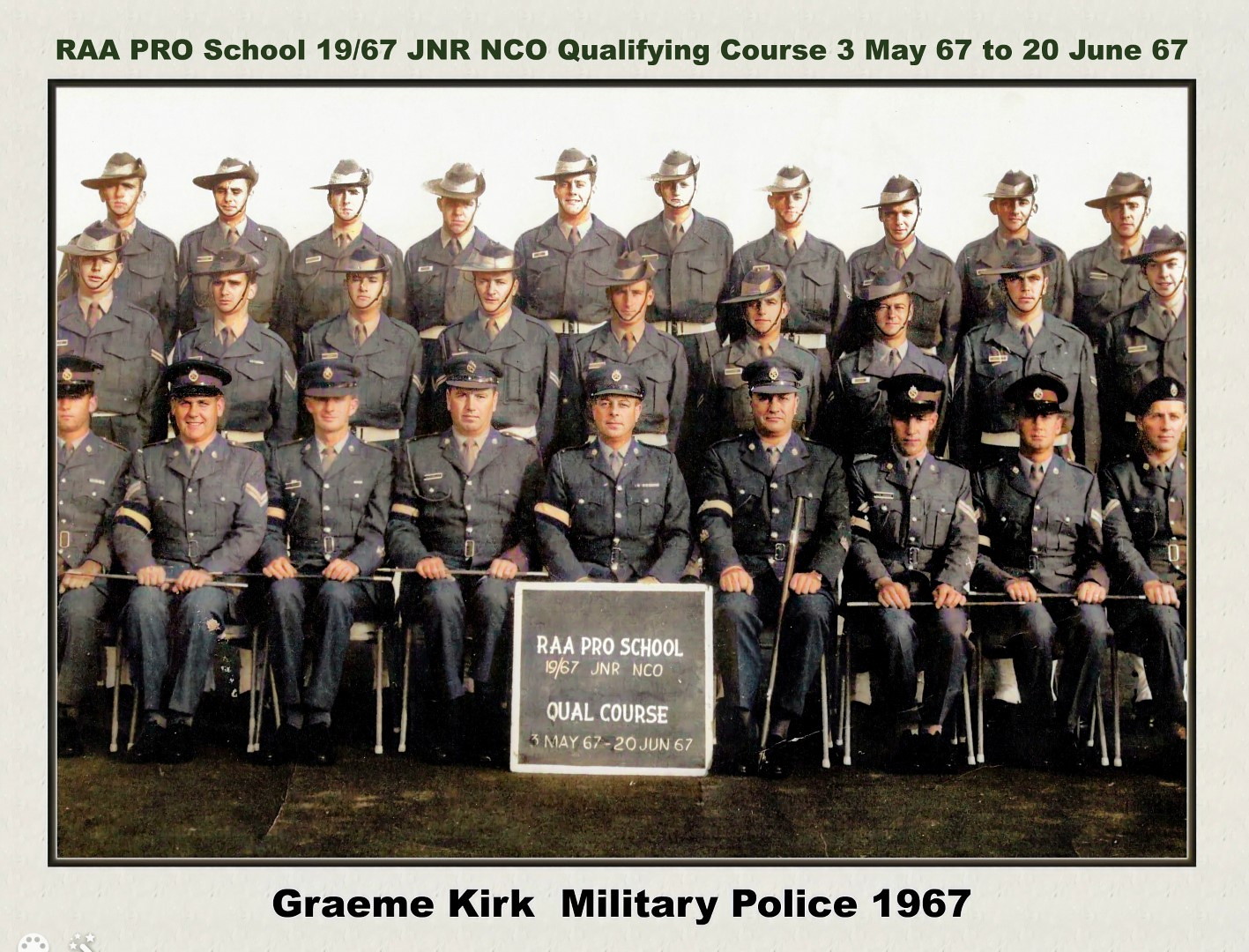The colorized photo from 1967 captures a formal gathering of about three dozen military police, posing against a white background with a drab brown floor. The group is divided into three rows, with the front row seated, appearing to be higher-ranking officers distinguished by their decorative uniforms and hats, while the back rows resemble privates in gray military garb. Centrally positioned in the front row is a sign leaning against a seated officer, reading "RAA Pro School 1967 JNR NCO Qual Course 3 May 67 to 20 June 67." The top of the image bears the same text, further framing the significance of the event. At the bottom, a caption states, “Graham Kirk Military Police 1967,” adding to the historical context.